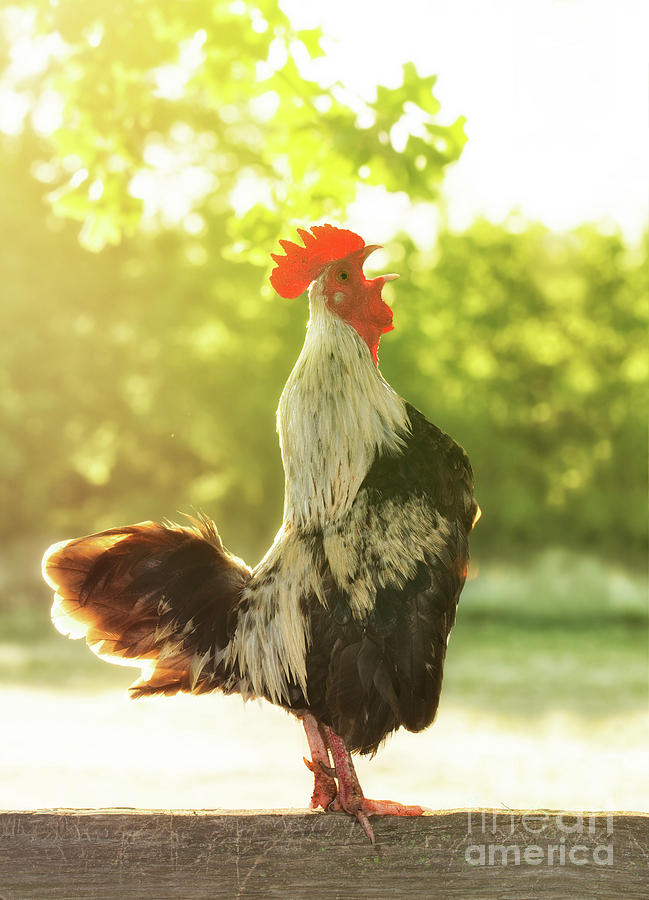In this detailed portrait-mode photograph by Fine Art America, a rooster stands tall on a wooden fence piece, set against a backdrop of early morning light filtering through blurry trees. The rooster’s beak is wide open, exuding a sense of greeting the dawn. Its vibrant red comb and wattles contrast strikingly with its off-white neck feathers, while its body features rich brown plumage, including the tail feathers. The rooster’s legs are a vivid orange color, indicative of its rural, farm-like setting. The lower right corner of the image bears the Fine Art America watermark, subtly acknowledging the source of this captivating rural scene.